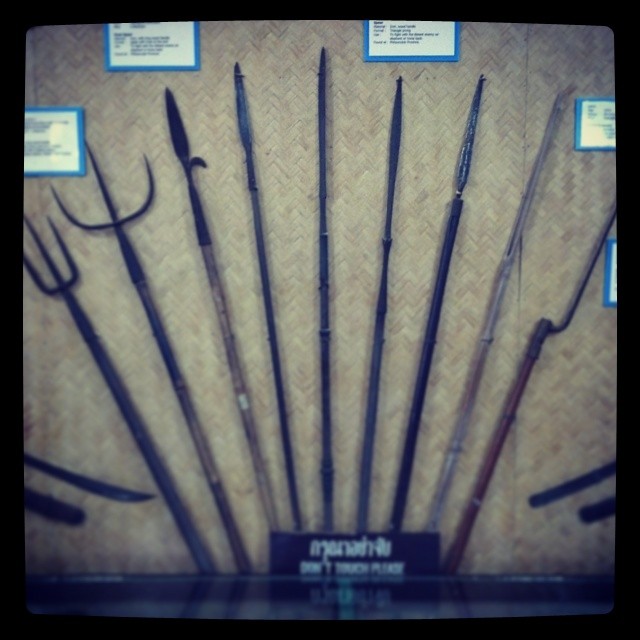The image features a collection of medieval tools or weapons, displayed against a woven beige background resembling a rattan or straw material, likely within a shadowbox or display case. The photo is slightly blurred, making it difficult to discern finer details. There are about nine tools, each with its own type and design. On the far left is a long fork-like tool with a black handle and three prongs. Next to it is a long black post with a curved, half-circle pointy end. Further along is a black and brown rod with a rounded spear-like tip, followed by a longer black rod that thickens slightly at the tip. Progressing rightward, there are three thin black rods, one of which has a shiny separator towards its top. Another item resembles a rod made from brown bamboo. The final tool on the right features a brown base with a top that loops up but is slightly cut off in the image. Small white labels with blue borders and black writing are placed intermittently among the tools, though the poor photo quality renders them unreadable. Additionally, there are two small black, pointy knife-like tools at the far left and far right at the bottom of the display. A black label with white writing is positioned at the bottom center, but it too is unreadable due to the blur.